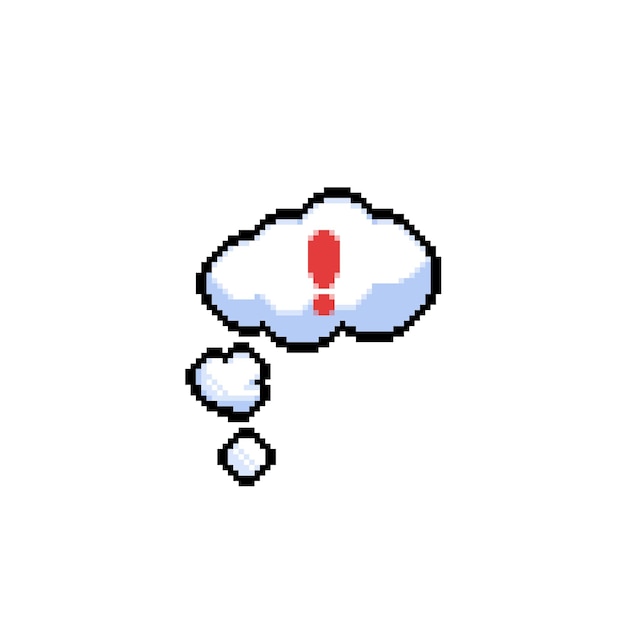The image features a pixelated, arcade-like graphic on a white background, resembling a three-part thought balloon. At the top, the largest section is a cartoonish Cumulus cloud with a thick black outline, white at the top, and light blue shading along the bottom. Prominently displayed in the center of this cloud is a bright red exclamation point. Below this primary cloud, there are two smaller puff-like shapes, also outlined in black. The middle shape, somewhat resembling a heart or blob, and the lowest shape, looking almost like a circle, both share the same white interior with blue shading. The entire graphic, characterized by its pixelated style, suggests a thought or conversation bubble.